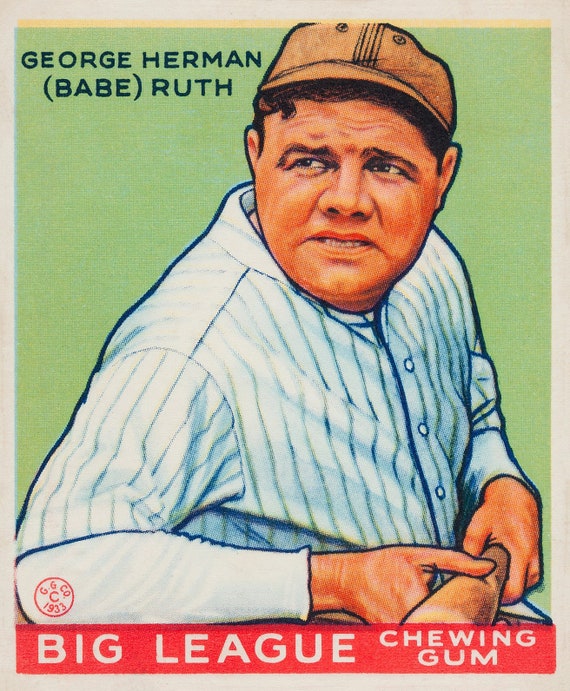This early 1900s vintage baseball card, possibly an advertisement or a label for Big League Chewing Gum, features a colorized drawing of the legendary Babe Ruth. Displayed from his head to his waist, Babe Ruth is captured mid-pose in his iconic pinstriped Yankee uniform and a brown baseball cap. The cap bears no logo, and his short dark hair is visible beneath it. A side view of Babe Ruth shows him holding a baseball bat across his stomach, conveying a slight grimace as if from the day's exertions. The background of the image is light green, enhancing the realistic but not photorealistic portrayal. In the top left corner, the text reads "George Herman (Babe Ruth)," while at the bottom, a red stripe with white lettering announces "Big League Chewing Gum." Additionally, the card features a small circle with text indicating "G.G.C.O. 1933," marking its vintage authenticity.